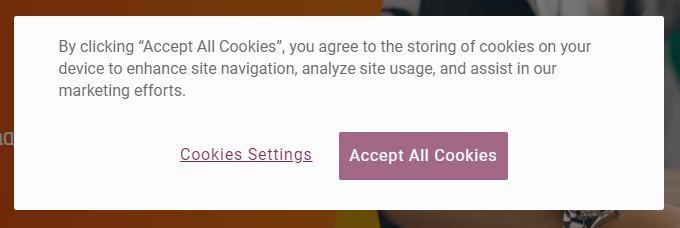Screenshot of a website in landscape mode, featuring a prominent cookie consent notification. The notification is displayed within a white, hard-edged text box that contrasts against a colorful background. The text within the box is gray and reads: "By clicking 'Accept All Cookies,' you agree to the storing of cookies on your device to enhance site navigation, analyze site usage, and assist in our marketing efforts." 

At the bottom of the text box, on the left side, there is an underlined "Cookies Settings" option in pink text. On the right side, a pink button with white text states "Accept All Cookies." The background of the notification has an interesting color division: the left-hand side features a solid block of orange with possible white text or symbols, while the right-hand side consists of shades of gray and possible skin tones. The overall design is minimalist and corporate, with no additional visual flair or subtle details beyond the straightforward notification and vibrant, divided background.